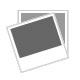This is a color photograph taken inside a house, focusing on an elegant display set on a table with a beige, slightly wrinkled tablecloth. Centered on the table are eight intricately designed silver goblets, exhibiting raised Greco-Roman patterns of roses and olive vines. The goblets are arranged in rows of four and dominate the central focus of the image. On the far left side of the table, partially cropped out, is a matching silver teapot with similarly elaborate designs. In the background, a wooden chair can be seen against a window. The view through the window shows a snowy yard adorned with trees, a birdhouse, and a glimpse of a house across the road. The angle of the photograph is slightly downward, adding to the ornate and slightly whimsical presentation of the scene.